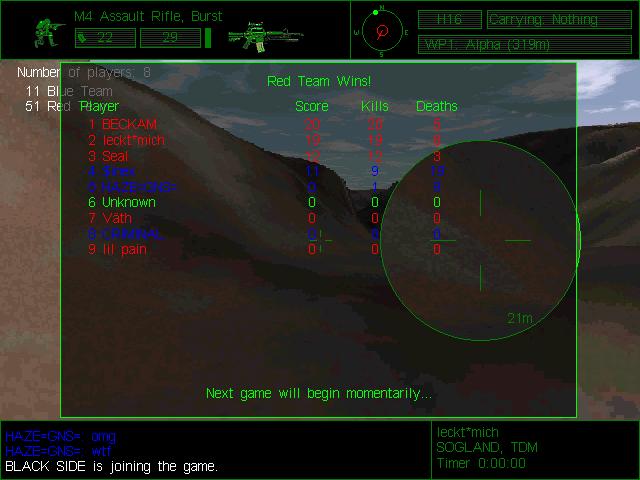This photograph captures a computer screen displaying an in-progress video game. The top and bottom of the screen feature a black thick border, with no such borders on the sides. At the top, green text announces "Red Team Wins," accompanied by the statement "Next game will begin momentarily" at the bottom. The lower portion of the screen also features white text reading "Black side is joining the game," alongside other elements, including "Sogland TDM" and a timer.

The gameplay occurs in a desert-like, mountainous environment. The mountain extends from the top left, dips in the middle, and rises again towards the right, beneath a blue sky adorned with white clouds. Within the game display, a green square frames the live in-game action, central to the screen.

Player names, scores, kills, and deaths populate the upper left side, suggesting it's a leaderboard or score summary. A prominent circle on the right side lists stats such as score, kills, and deaths near the screen's center. The top also showcases "M4 assault rifle burst," indicating a weapon, with a small depiction of a squatting player holding a gun. Further to the right, there's a compass and additional text like "carrying nothing" and "alpha." The interface includes various text colors—green dominates, punctuated by red and royal blue texts, with some white text elements. Lastly, a crosshairs graphic implies the targeting mechanism in the game.